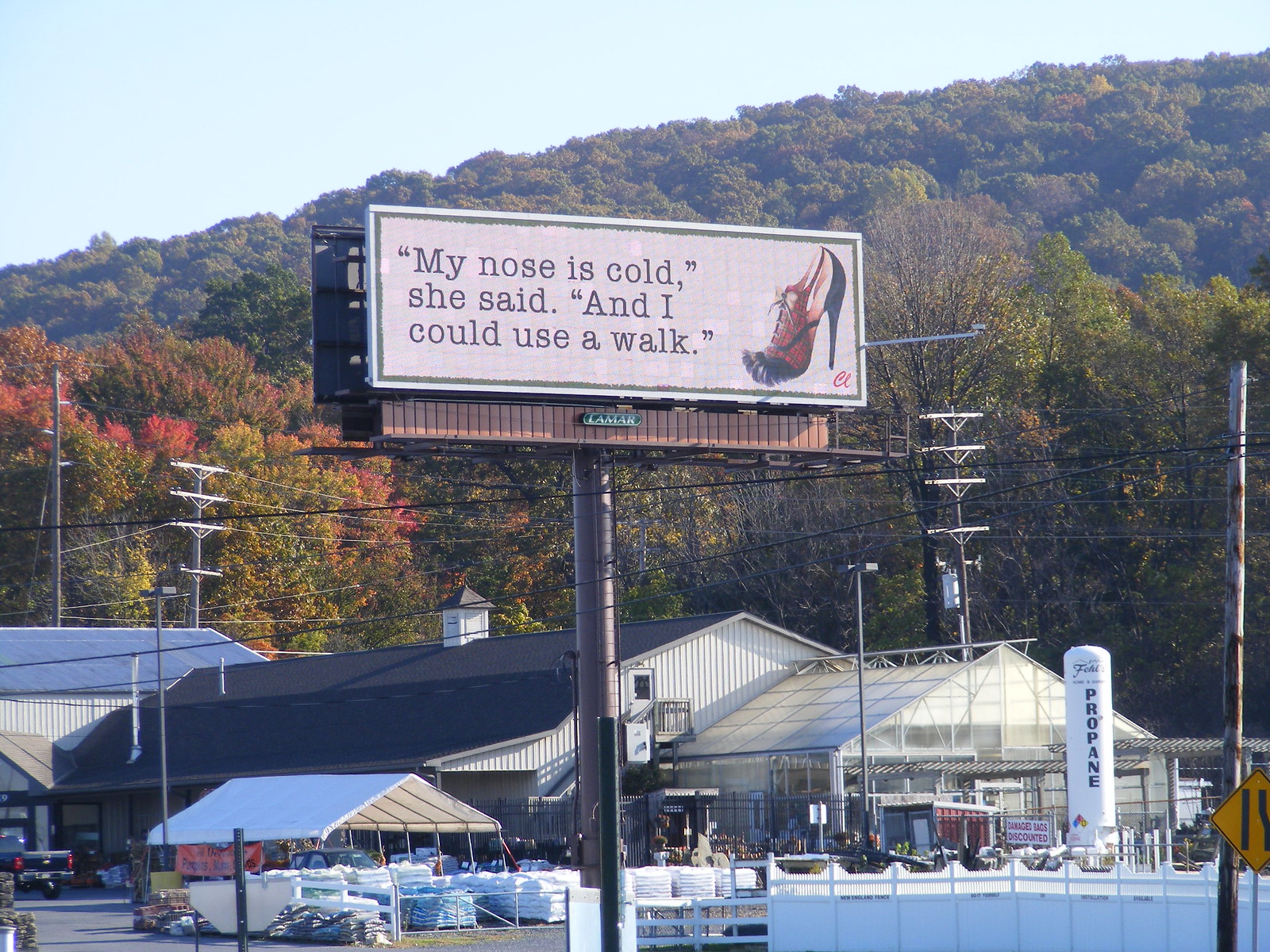The photograph captures an outdoor scene dominated by a market store with a home and garden center aesthetic. The store exhibits barn-like architecture, featuring a greenhouse with a glass construction at one end. Parked cars, pallets of goods, and stacks under a tent can be seen in front of the store. The backdrop displays a picturesque hill covered in trees, many of which are transitioning into autumn with a mix of green, red, and yellow leaves. Above it all, the sky is a bright, light blue.

Central to the image is a prominent billboard elevated on a large brown pole, situated by the roadside. The billboard has a light tan background with brown lettering that reads, "My nose is cold, she said, and I could use a walk," on the left-hand side. The right-hand side showcases a high-heeled stiletto shoe, stylized and striking. Below the billboard, a large white cylindrical propane tank with a warning sign is visible, emphasizing the practical nature of the market. Additionally, a yellow road sign indicates merging lanes, and telephone lines crisscross the scene, adding to the blend of commercial and natural elements.